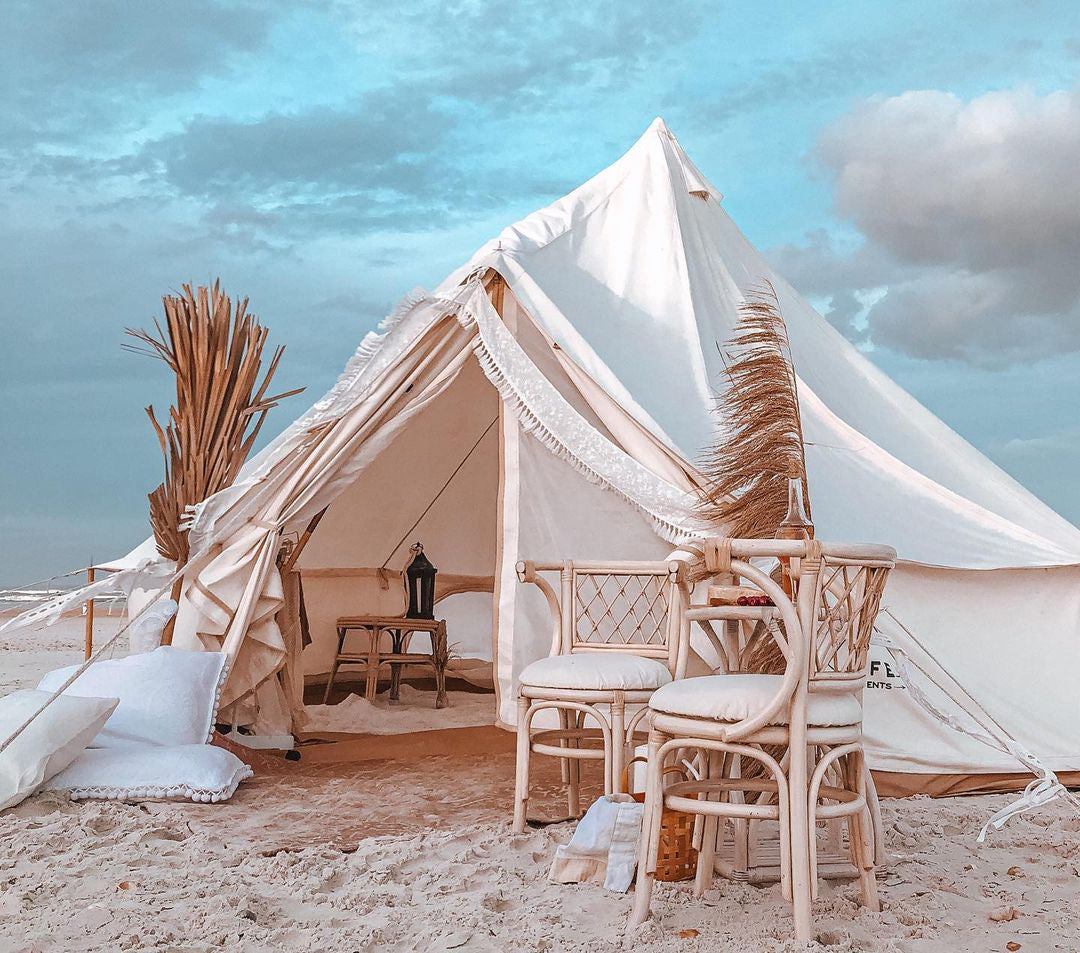The image captures an outdoor scene featuring a glamping setup on a sandy beach. At the center is a spacious white canvas tent with walls that rise a few feet before angling upwards to meet at a central pole. The tent's front is open, revealing an interior with a wooden brown coffee table, some rugs, and a ventilation window. Hanging over the doorway are decorative tassels, adding a cozy touch. The tent sits on fine, tan-colored sand, sprinkled with leaves. Outside the tent, on the right side, are two wicker-like chairs in a light or white color, along with a small table bearing a wine glass and bottle. On the left of the door, there are a couple of white pillows and tassels, as well as a palm broom. A glimpse of the ocean is visible in the background to the left, while the sky above is a mix of light blue and patchy white clouds, transitioning to a more grayish hue towards the bottom. This picturesque setup, nestled in white or very light sand, suggests an inviting and serene glamping retreat.